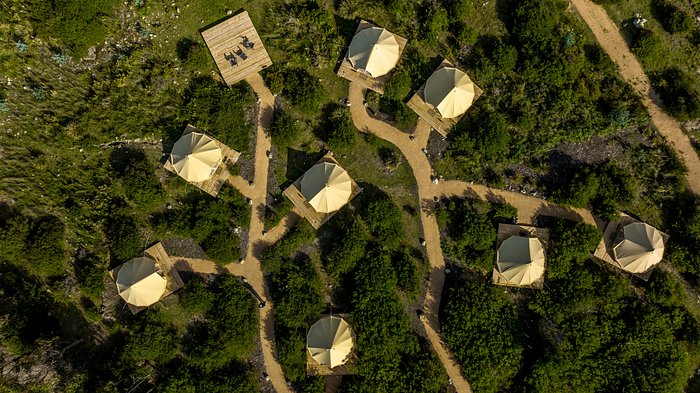This top-down aerial photograph captures a lush, green residential neighborhood or vacation village, characterized by eight circular, white canvas-roofed structures that resemble teepees or unique style homes. These structures are arranged in a seemingly haphazard manner amidst dense foliage and green fields, connected by a network of dirt roads and pathways. A prominent feature in the image is a dock located at the top, adorned with three beach chairs, suggesting a relaxing spot by the water. The dirt road diagonally cuts through the left side of the scene, while multiple trees and green spaces are interspersed between the clustered dwellings. The light source appears to be coming from the right, casting natural highlights across the tranquil environment.